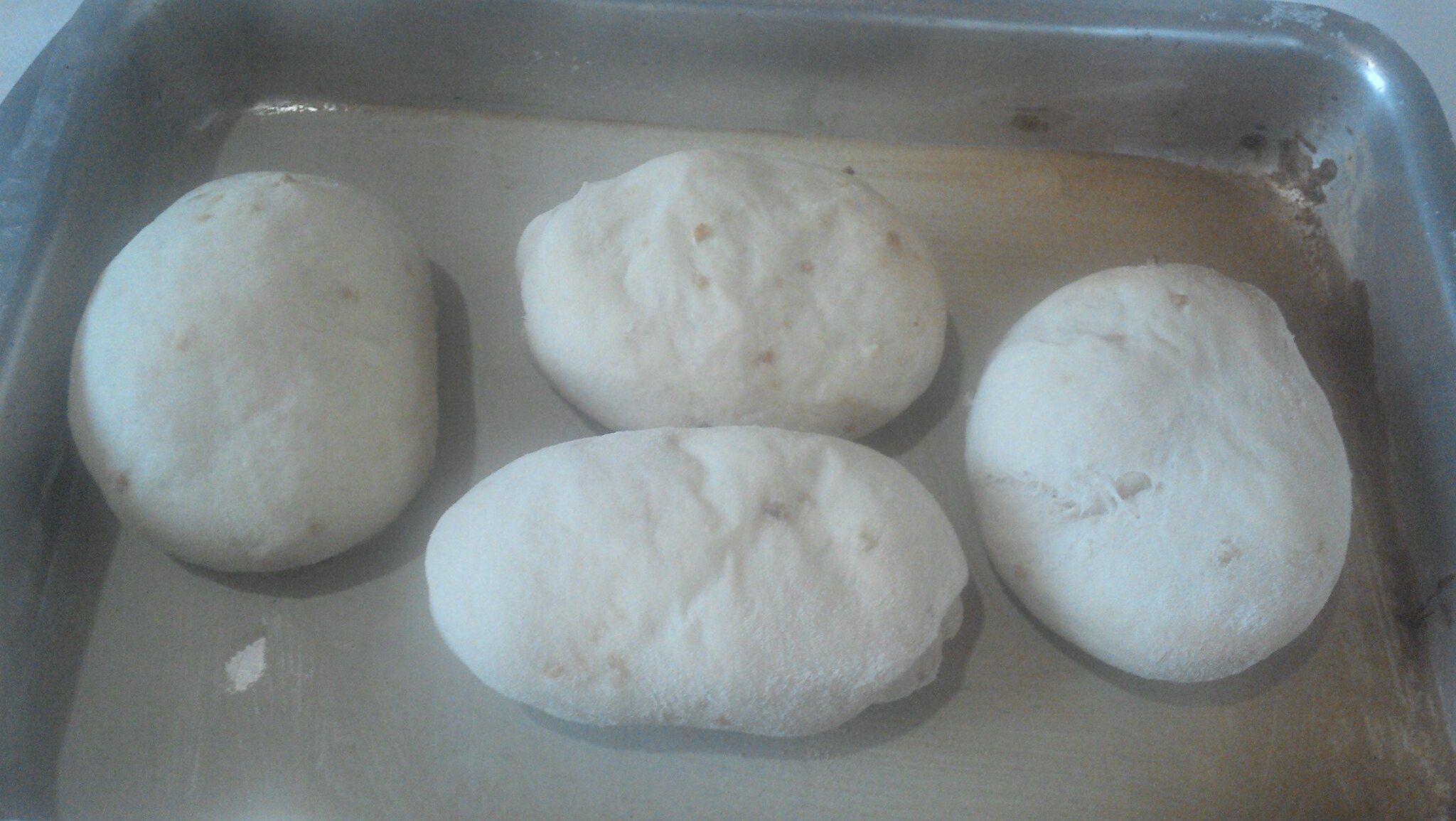This photograph captures a close-up view of a well-weathered, silver rectangular baking pan, greased with a brownish-yellowish tint. The pan contains four large, ovular dough balls, aligned lengthwise to the camera. The white dough, with subtle brown imperfections, appears uncooked and ready for baking. The dough balls are positioned with one at each end and two in the middle, slightly touching each other. The image is slightly blurry, possibly due to steam or smoke in the kitchen, indicating that other cooking activities might be taking place.